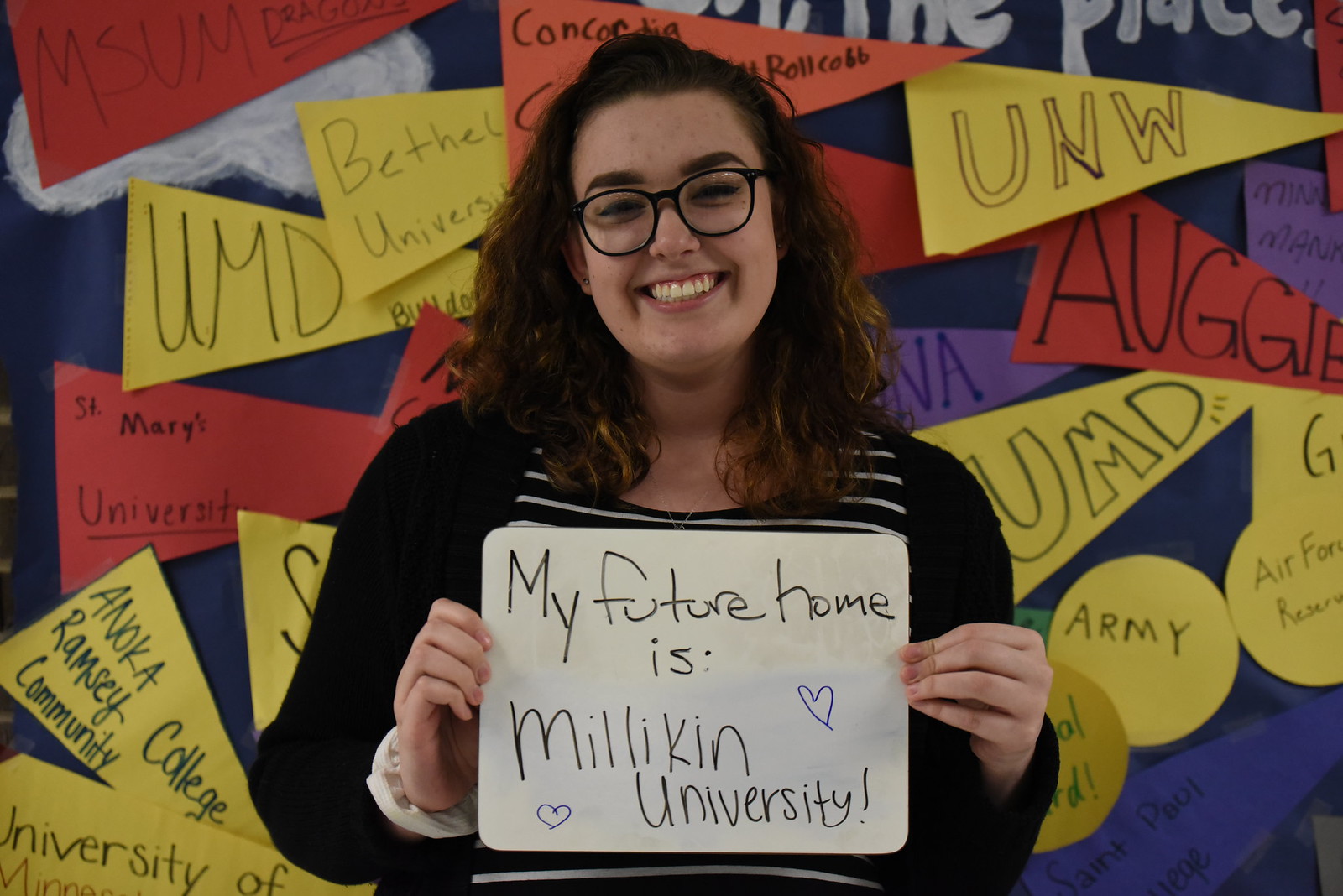A young woman, likely in her late teens or early 20s, stands smiling at the camera. She has brown, wavy, shoulder-length hair, partially pulled up, and she wears black glasses that frame her expressive, thick eyebrows. Her outfit consists of a black cardigan over a black and white striped shirt. In her hands, she holds a small whiteboard, about a foot across, positioned in front of her chest. Written in black marker on the whiteboard are the words, "My future home is Milliken University," accompanied by two blue hearts drawn on either side of the university's name. 

The backdrop consists of a blue or purple wall adorned with various triangular and circular banners. These banners represent different universities and colleges, including UMD, UNW, Augie, Bethel University, and Anoka-Ramsey Community College, as well as signs for the Army and Air Force Reserves, suggesting a strong college-preparatory atmosphere.